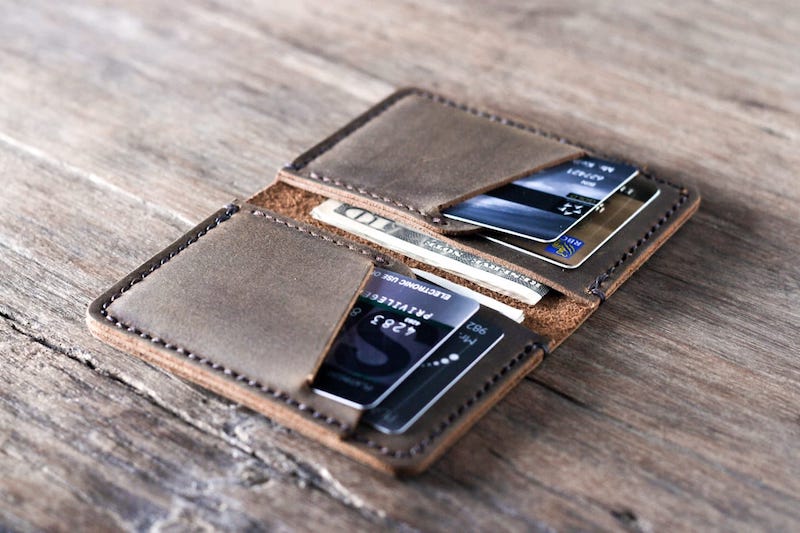In this detailed close-up photograph, an open brown leather wallet, complete with meticulous stitching, rests on a medium-toned, unfinished rugged wooden table. The wood surface, displaying natural hardwood grain and some signs of wear such as debris and cracks, complements the wallet’s rustic aesthetic.

The wallet is distinctly non-traditional with two halves, each harboring two credit card slots. On the left side, one card is primarily cyan or mid-blue, gradating to dark blue, with another dark blue card beneath it. The right side reveals a brown card with dark blue at the top and another card featuring a gradation from dark blue to white then back to different shades of blue. Additionally, within this half, there’s a crisp, folded US $10 bill, clearly visible, signifying some stored cash, while the left side hints at the possibility of more money tucked away.

This photograph captures the essence of a well-used but well-maintained man’s wallet, juxtaposed against a similarly rugged and storied wooden table, providing a harmonious composition of textures and colors.